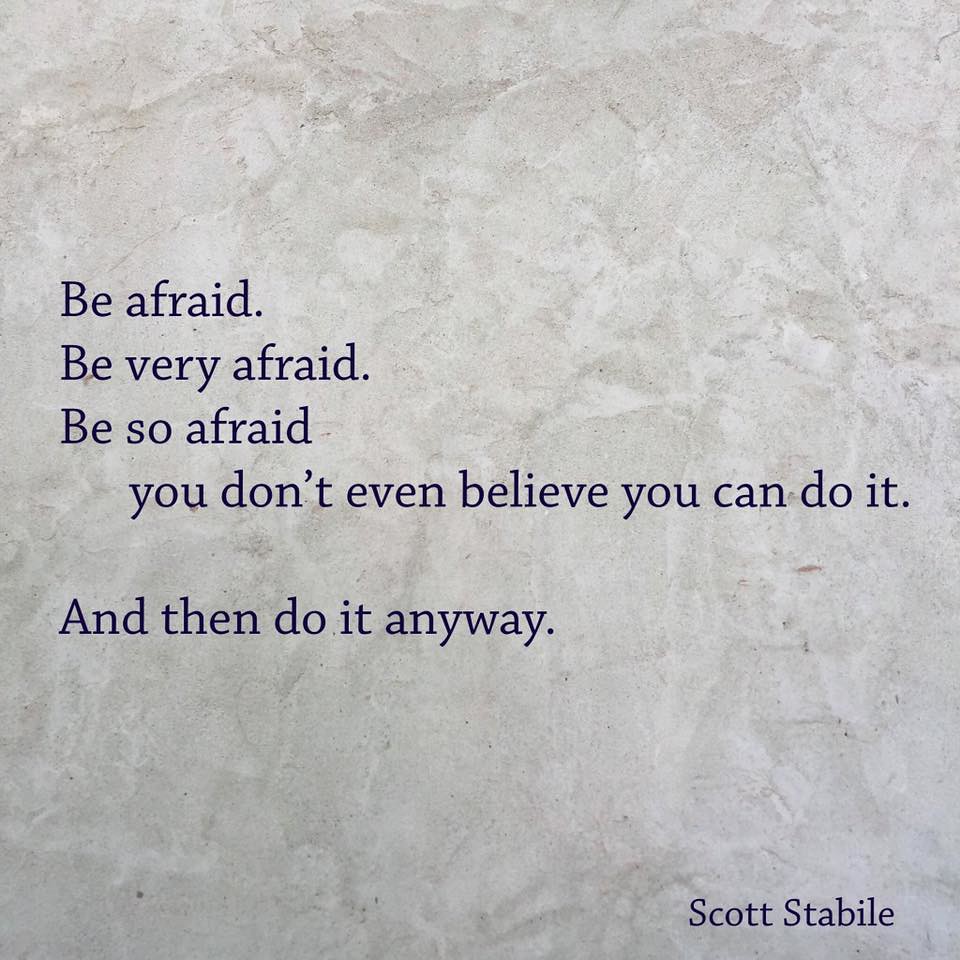The image is a large square featuring a marbled background in shades of white and brown, giving it a rugged, textured appearance reminiscent of watercolor or crumpled paper. Dominating the middle portion of the image is left-aligned black text that reads: "Be afraid. Be very afraid. Be so afraid you don't even believe you can do it, period. And then do it anyway." In the bottom right corner, the name Scott Stabile, spelled S-T-A-B-I-L-E, is present, indicating the author of the inspiring and motivational quote. The overall aesthetic hints at a blend of vulnerability and resilience, encouraging viewers to face their fears and persevere.